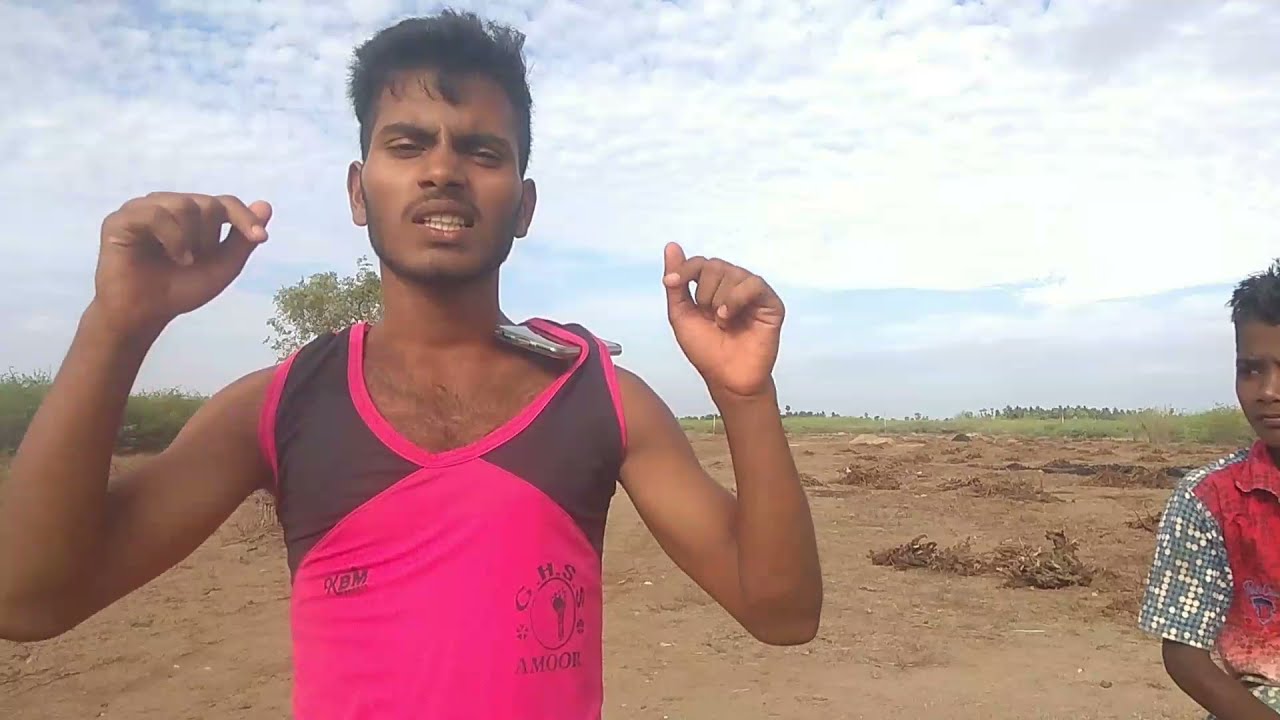In this landscape-oriented color photograph, a central figure, likely in his late teens or early twenties, is prominently positioned on the left side of the image, facing the viewer with both hands raised near his jawline as if he is in mid-conversation or explaining something. This dark-skinned man, potentially of Middle Eastern or Indian descent, sports a crew cut with bangs grazing midway down his forehead. His eyes are slightly squinted and his mouth is open, revealing both his upper and lower teeth. A thin mustache and beard frame his expressive face. He is wearing a sleeveless tank top that is predominantly bright pink with a black shoulder section and text on it, including "AMOR" at the bottom. A noticeable detail is his cell phone, which is tucked under the edge of his tank top on the right side. 

To the far right of the image stands another young boy, roughly between 12 to 15 years old, also dark-skinned with dark hair. He gazes up at the main figure, dressed in a shiny, red shirt that transitions into pink, with speckles of gray and yellow dots adorning the sleeves and upper portion. 

The background features a vivid setting of light-colored clouds dotting the sky. The ground is mostly dirt, stretching out to a distant line of trees and scattered vegetation, adding depth to the scene.